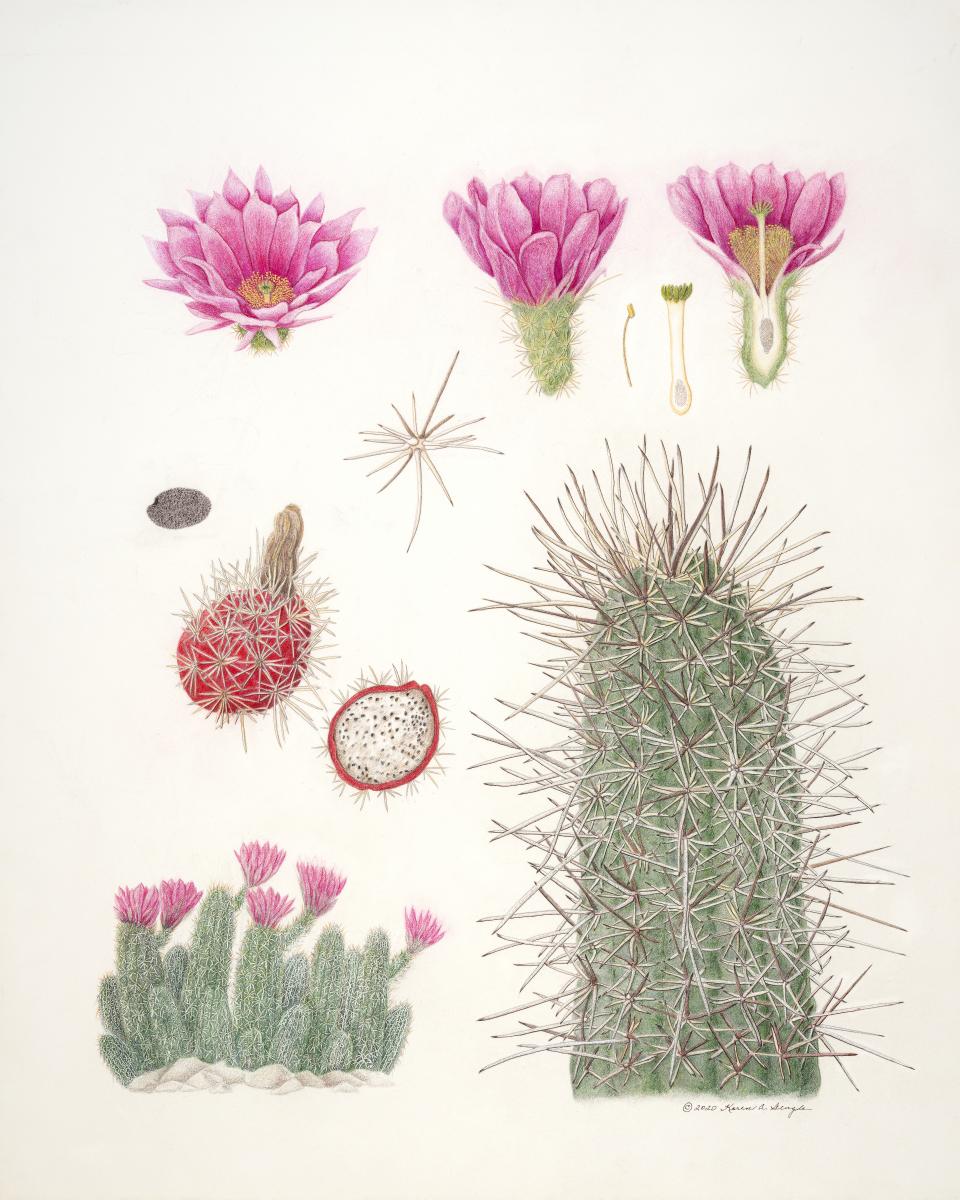This detailed illustration, reminiscent of an older textbook or classroom poster, meticulously breaks down the anatomy of a specific cactus species on a white background. The central image showcases a green cactus bristling with spines, each quill drawn with painstaking detail, suggesting the use of colored pencils. At the top of the poster, three vibrant pink cactus flowers are depicted in various stages of bloom, their petals meticulously displayed. Adjacent images offer a closer examination: a vertically cut flower revealing its internal structure, and red bulbous seed pods, one intact and another halved to disclose the seeds within. The bottom left portion of the illustration portrays a cluster of green cacti, adorned with pink flower buds sprouting upwards, all rooted in a rocky terrain. This composition is further authenticated by an artist’s signature in the lower right corner, reinforcing its illustrative and educational value.